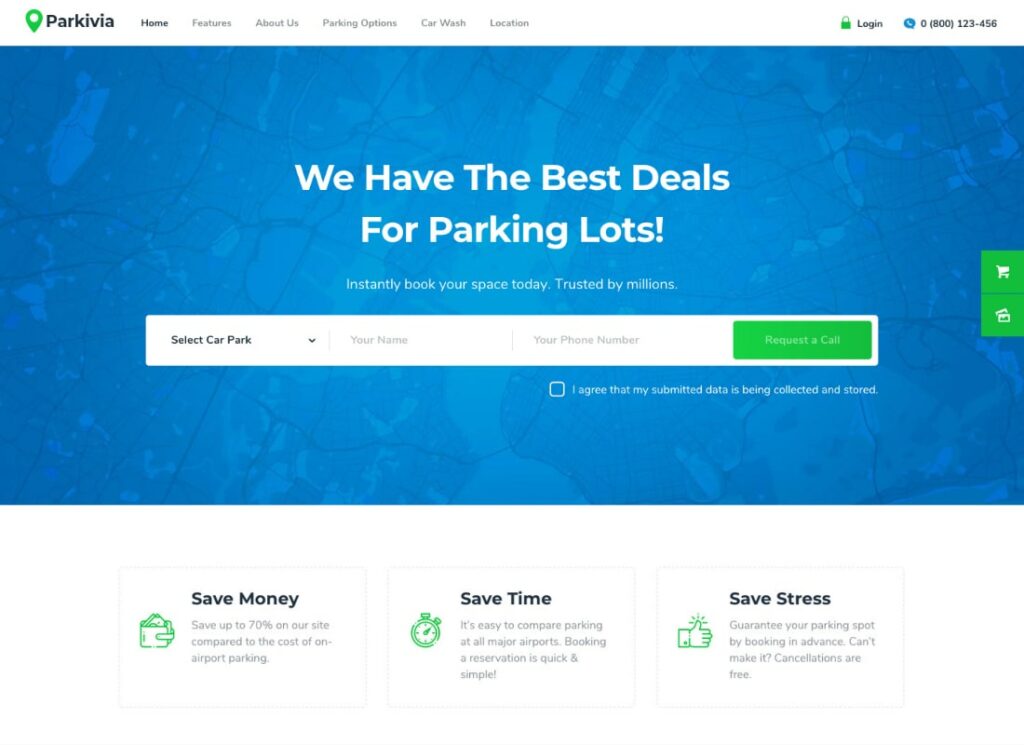The screenshot displays an interface for Park Viva, featuring a translucent blue overlay revealing a map underneath. Prominently, in bold white text, it states, "We have the best deals for parking." The navigation menu includes fields for selecting a car, entering your name, and your phone number. A green button labeled "Request a Call" is available alongside a checkbox that reads, "I agree that my submitted data is being collected and stored." 

Additionally, there are two solid green boxes: one with a white shopping cart icon and another indicating tickets. Below, three white boxes showcase the benefits of using Park Viva, each highlighted with green icons and labeled "Save Money," "Save Time," and "Save Stress."